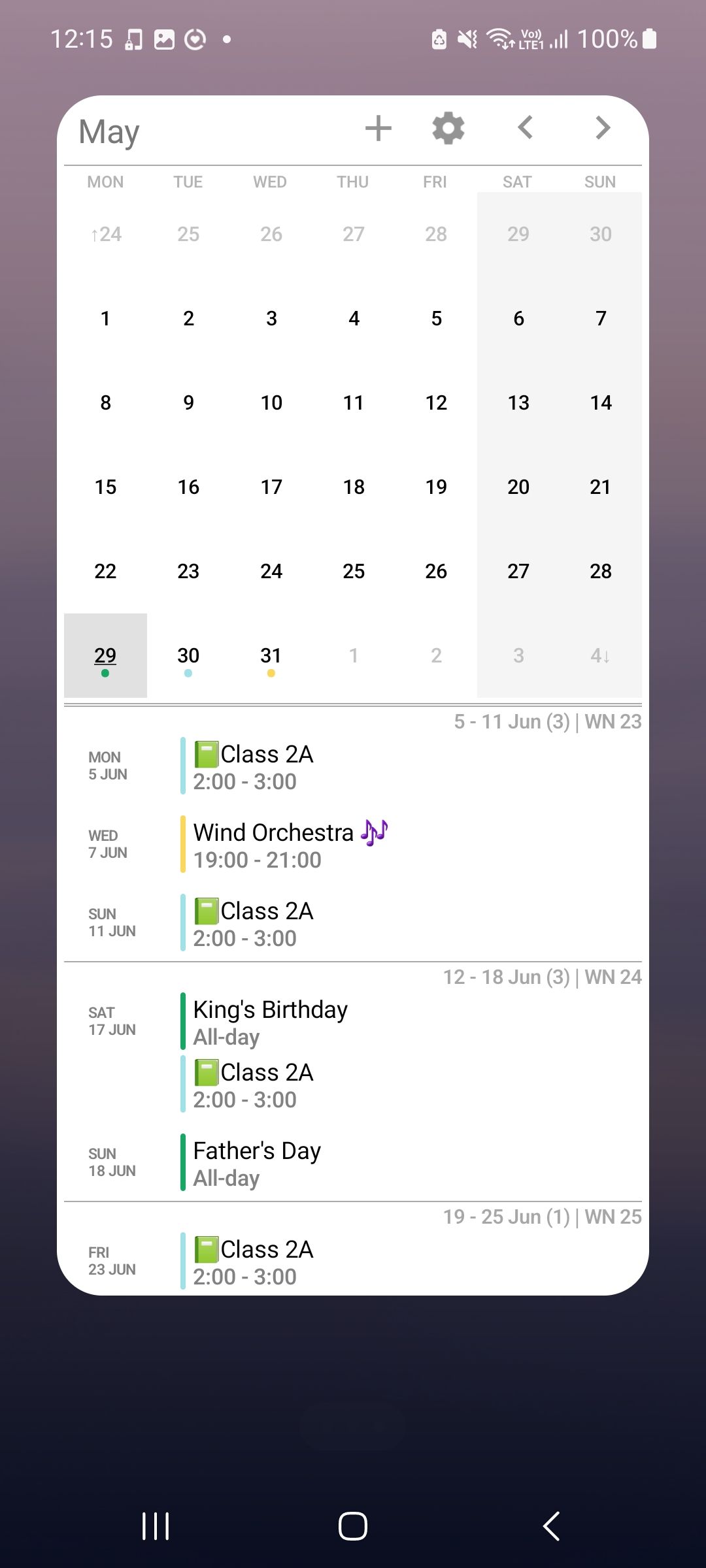This image appears to be a highly detailed calendar or schedule, displaying various events and information. 

At the top center, the image reads "1215." Directly beneath this title, a strong visual representation can be seen, featuring an icon of a hard receiver or perhaps a speaker. Adjacent to this is a symbol for full Wi-Fi signal strength, indicating 100% connectivity. Flanking these symbols on both sides are gear icons, suggesting settings or configurations.

The calendar is organized into rows by days of the week: Monday, Tuesday, Wednesday, Thursday, Friday, Saturday, and Sunday. 

Below the days of the week, the calendar is populated with numerous dates and events:
- Each day is shown with a number, spanning from 1 to 31.
- Specific events are noted, such as "Class 2A" occurring daily from 2 to 3 PM.
- Key dates include:
  - Monday: King's Birthday (All Day)
  - Father's Day: All Day
  - Wind Orchestra: 19th to 21st
  - Monday (5th June), Wednesday (7th June), Sunday (11th June), Saturday (17th June), Sunday (18th June), Friday (29th June)

At the bottom of the calendar, the visual detailing includes an amber domain square followed by a dot, which transitions into a sideways arrow. This section appears to be highlighted in white, potentially to draw attention or signify importance.